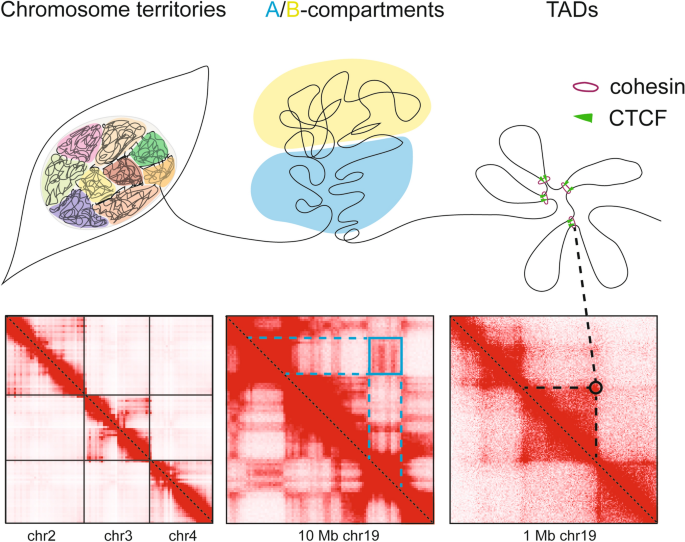This detailed scientific illustration, possibly from a textbook, vividly depicts the concept of "Chromosome Territories" against a white background. At the top, the heading "Chromosome Territories" introduces the image. Directly beneath, interconnected with a line, is a second heading labeled "A/B Compartments," where 'A' is depicted in blue and 'B' in yellow. This section represents the organization of chromosomes into different territories and compartments within the nucleus. 

Following a linear progression from left to right, the illustration elaborates on how chromosomes unwind, transitioning into regions labeled "TADs" (Topologically Associating Domains) with further annotations "Cohesion" and "CTCF" indicating key proteins involved in the chromatin structure.

At the bottom right, the illustration features a square image resembling a microscopic or radiological interpretation with a diagonal line and the text "1MbCHR19" in red on a white background. Adjacent to it, moving leftward, is a more intricate diagram marked by dotted blue lines, with another diagonal line annotated "10MbCHR19."

The final square image on the bottom left displays a clear, nine-space grid. This detailed segment includes a red-stained microscopic or radiology image with a diagonal dotted line, and black text labels "CHR2," "CHR3," and "CHR4," correlating to chromosome territories, A/B compartments, TADs, Cohesion, and CTCF. The extensive use of color and detailed annotations make the illustration an informative depiction of the spatial organization within the nucleus.